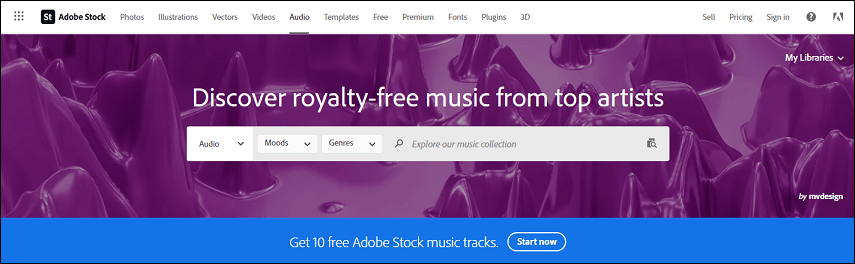The image depicts the Adobe Stock website, featuring a clean and organized user interface. The top menu is housed within a white bar, prominently displaying a dotted 3x3 cube icon followed by a black box with the initials "ST." Adjacent to this, "Adobe Stock" is highlighted in bold black letters. The menu options are neatly laid out, starting with Photos, Illustrations, Vectors, Video, and Audio, the latter of which is currently highlighted. Continuing in sequence are Templates, Free, Premium, Fonts, Plugin, and 3D. A slight gap separates these options from the final three: Sell, Pricing, and Sign In. An information button and the Adobe logo are also present in this section.

Situated below this navigation bar is a vivid purple abstract painting serving as a background. Overlaying this artwork in bold white letters is the headline: "Discover Royalty-Free Music from Top Artists." Beneath the headline, there are interactive search options labeled Audio, Moods, Genre, and a Search button with a magnifying glass icon accompanied by the text "Explore Our Music Collection."

In the same purple section, the top right corner features "My Libraries" with a dropdown menu, and at the bottom right, the phrase "Buy My Design." Below this is a striking blue box that offers "Get 10 Free Adobe Stock Music Tracks," accompanied by a clickable "Start Now" link.